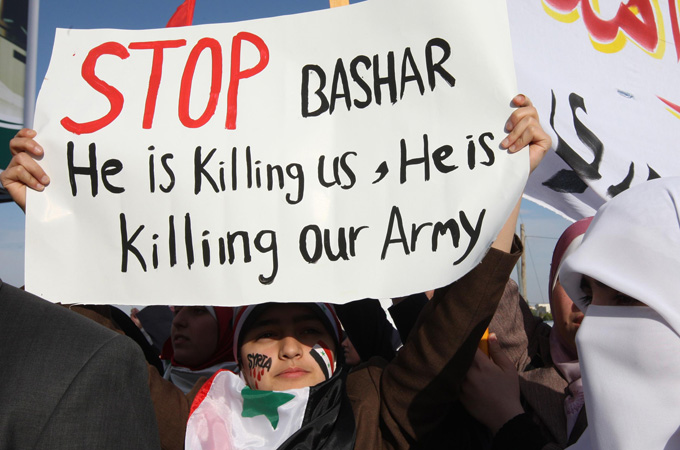In this image of a protest scene, a young woman with brown skin stands at the forefront, donning a black long-sleeve shirt or hoodie, and her head is covered with a hood or hat that casts a significant shadow over her face. She has face paint on her cheeks and is wearing a scarf around her neck in red, white, and black with a green star - resembling the flag of a Middle Eastern country, likely Syria. The woman is holding a large white piece of construction paper with the words "STOP" in bold red letters in the upper left corner, followed by "Bashar. He's killing us. He is killing our army" written in black. 

The protest appears to be taking place outdoors under a blue sky, visible in the upper left of the image, and the scene is bustling with people holding various protest signs. Some signs are in different languages, contributing to the crowded yet passionate atmosphere. On the right, another person’s head, completely covered in white fabric with just their eyes peeking out, is visible. The crowd includes many others, likely a mixture of men and women, dressed in traditional and contemporary attire, with more protest signs seen in the background, some featuring intricate designs and scripts.